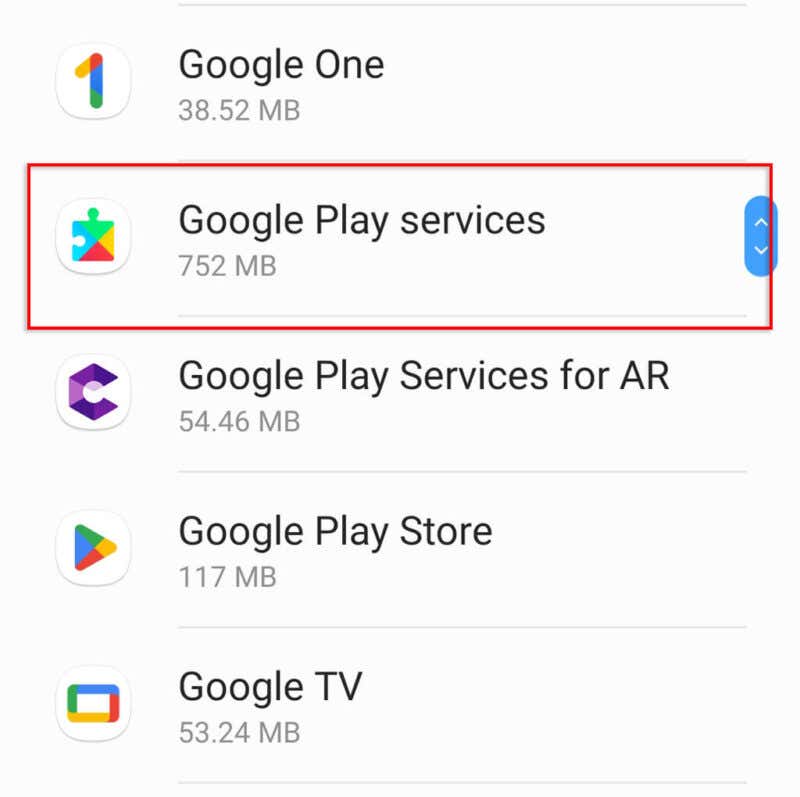This image features a white background divided into five vertical sections. Each section contains a distinct graphic on the left and corresponding text on the right.

1. **First Section**: At the top, there is a minimalistic line. Adjacent to it, on the left side, is a softly rounded square graphic composed of the colors yellow, red, blue, and green, forming the number "1." To the right, in black text, it reads "Google One" with both 'G' and 'O' capitalized. Beneath this, the size "38.52 MB" is specified.

2. **Second Section**: The second section mirrors the format of the first but features a softly rounded square with a puzzle piece in light blue, red, green, and yellow colors. Next to the graphic, the text "Google Play services" appears, with 'G' and 'P' capitalized. Below this, the storage size "752 MB" is noted. This section is accented with a red border.

3. **Third Section**: This part includes a purple 'C' encircling a softly rounded square. The text next to it reads "Google Play services for AR," highlighting the initials 'G,' 'P,' 'S,' and 'AR.' The size "54.46 MB" is listed beneath.

4. **Fourth Section**: The graphic here is another softly rounded square, this time containing a right-pointing triangle colored blue, red, green, and yellow. Accompanying this, the text states "Google Play Store," with 'G,' 'P,' and 'S' capitalized. The size "117 MB" is also mentioned below.

5. **Fifth Section**: In the final section, the graphic is a softly rounded square featuring an arrangement of green, yellow, blue, and red rectangles. The adjacent text reads "Google TV," capitalizing both 'G' and 'T.' Underneath, the storage size "53.24 MB" is specified. This section ends with a small line at the bottom.

Each section in the image provides detailed and colorful visual representations along with corresponding textual information, including application names and storage sizes.